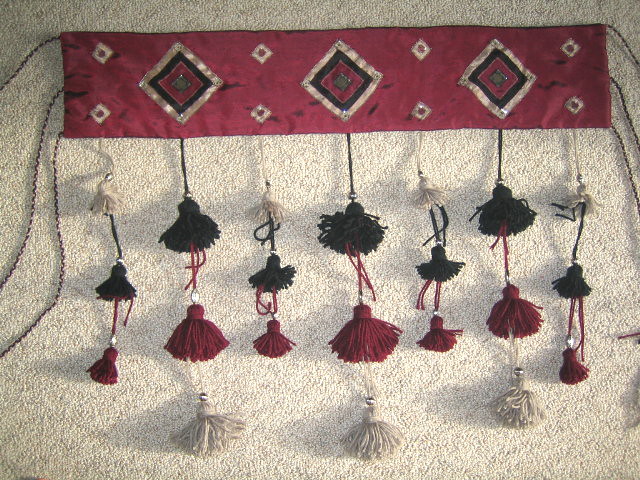The image depicts a landscape-oriented, detailed view of a richly adorned textile draped over a light beige carpet. At the top, a rectangular, shimmering red banner is prominently featured, embellished with a series of embroidered diamond shapes. The diamonds are organized in a pattern of alternating sizes—two small diamonds followed by a larger one—with each diamond displaying a sequence of colors: an outer silver stripe, followed by black, then red, and a small green diamond at the center. Each corner of these diamonds hosts tiny white diamond shapes with red dots in their centers, adding intricate detail to the design.

Three strings on each end of the banner dangle down the sides, suggesting it is designed to be tied or hung. Beneath the banner, seven tassels hang in a rhythmic pattern, characterized by their wool material and a sequence of colors—black on red on white—arranged in varying sizes from small to large. Each tassel is further segmented into three to four smaller fringe-like tassels with the colors gold, black, red, burgundy, and another black, burgundy, and gold repeating. Additionally, there are both small and larger pom-pom tassels that enhance the visual complexity and craftsmanship of the piece. This meticulously crafted fabric is presented against the soft, light background, highlighting its vibrant colors and intricate details.